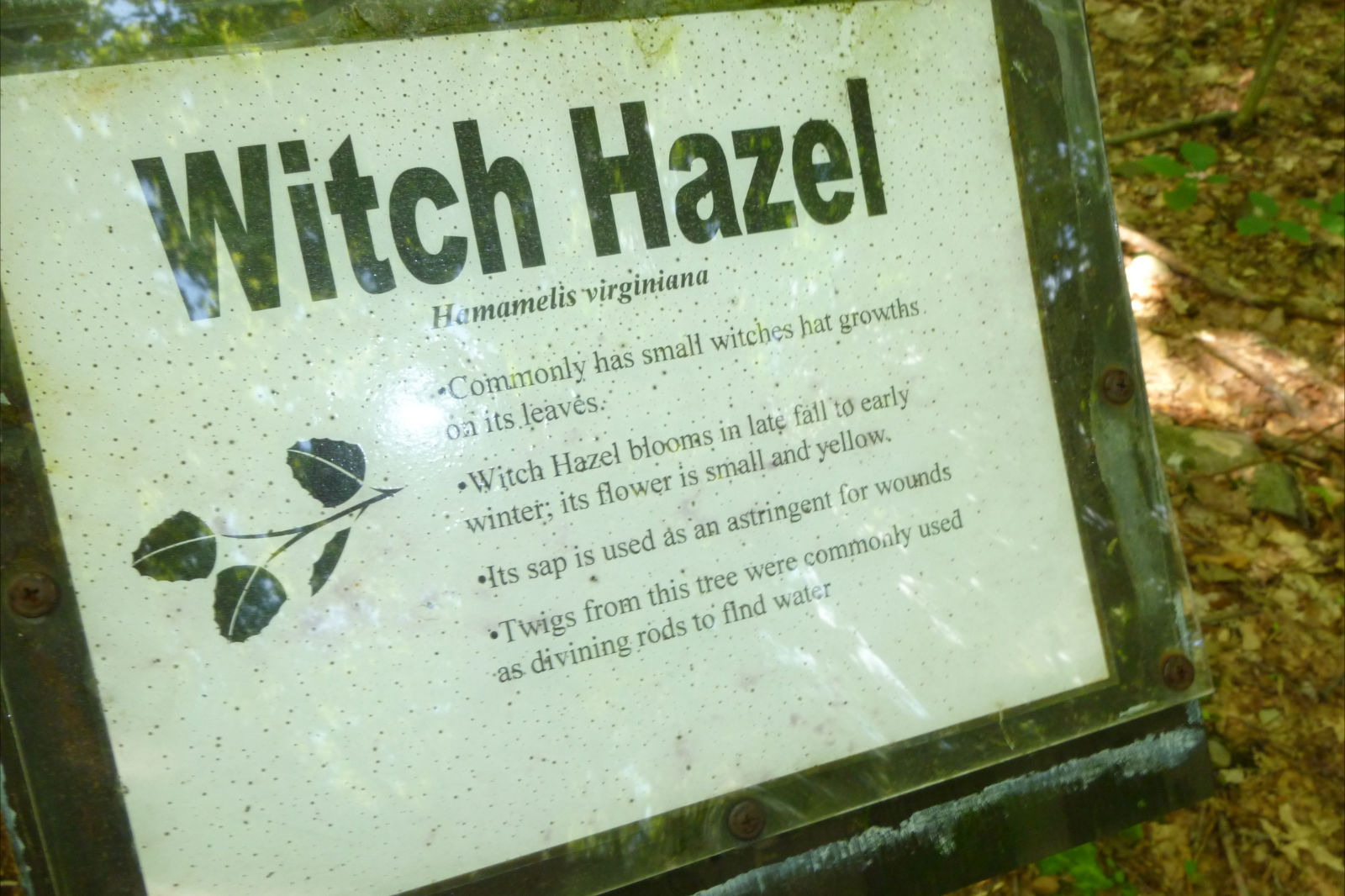The image captures an information plaque anchored in a wooded area, likely encountered during a hike. The plaque, framed by a black or dark border and covered with a weathered, dirt-flecked sheet of plexiglass secured by rusted screws, describes witch hazel. In black font, "Witch Hazel" is prominently displayed, followed by its Latin name, Hamamelis virginiana. Below, in Times New Roman 12-point font, it details that witch hazel commonly bears small, witch's hat-like growths on its leaves. The plant blooms from late fall to early winter, producing small yellow flowers. A depiction of greenish witch hazel leaves is also present. The text highlights practical uses for the plant, noting its sap’s astringent properties for wound care and the historical use of its twigs as divining rods to locate water. Sunlight filtering through the trees illuminates the leaves and ground around the plaque, enhancing the natural setting.